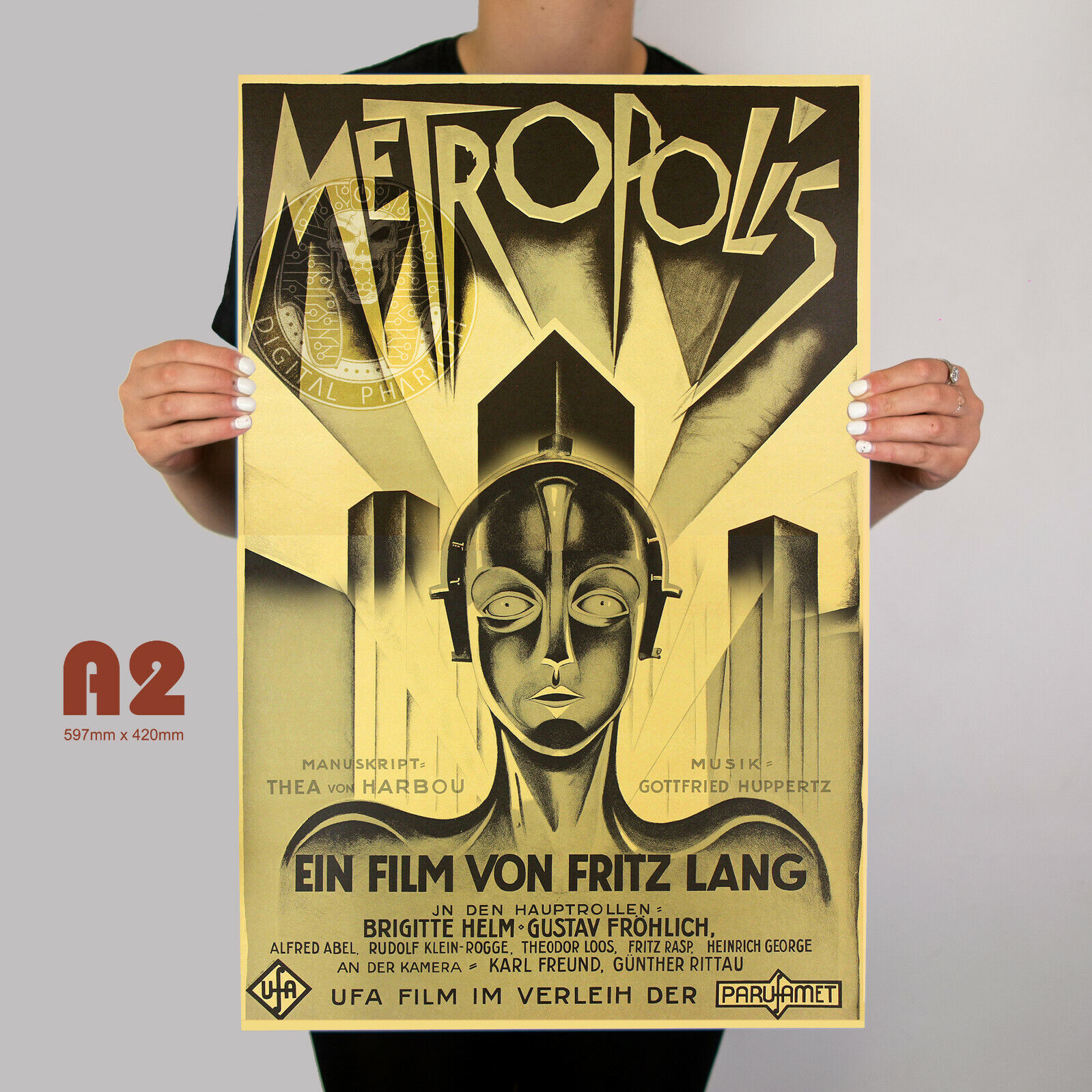In this detailed photograph, a woman stands against a grey-white background, holding a large, yellow and black movie poster. The woman’s head is cut off by the top of the photograph, and the image captures her from just above the neck to her knees. She wears rings on her fingers, and her nails are painted white. The poster, which she holds delicately by its edges, prominently features the title "Metropolis" in big, capital letters at the top, set against a black background.

The center of the poster displays a stylized illustration of a female robot with a futuristic and expressionless face, adorned with metallic headgear and large, blank eyes. The robot, depicted from shoulders to head, stands before a minimalist depiction of skyscrapers. 

Below the illustration, text reads "Ein Film von Fritz Lang," and additional credits in German include "Manuscript: Thea von Harbou" and "Music: Gottfried Huppertz" in grey font. A watermark resembling a stylized pharaoh with a skull face, encircled by the text "Digital Pharaoh," appears at the top left corner. A modern, dark red font near the bottom left of the photograph states "A2," with its dimensions "597mm by 420mm" noted beneath in a modest, simple font.